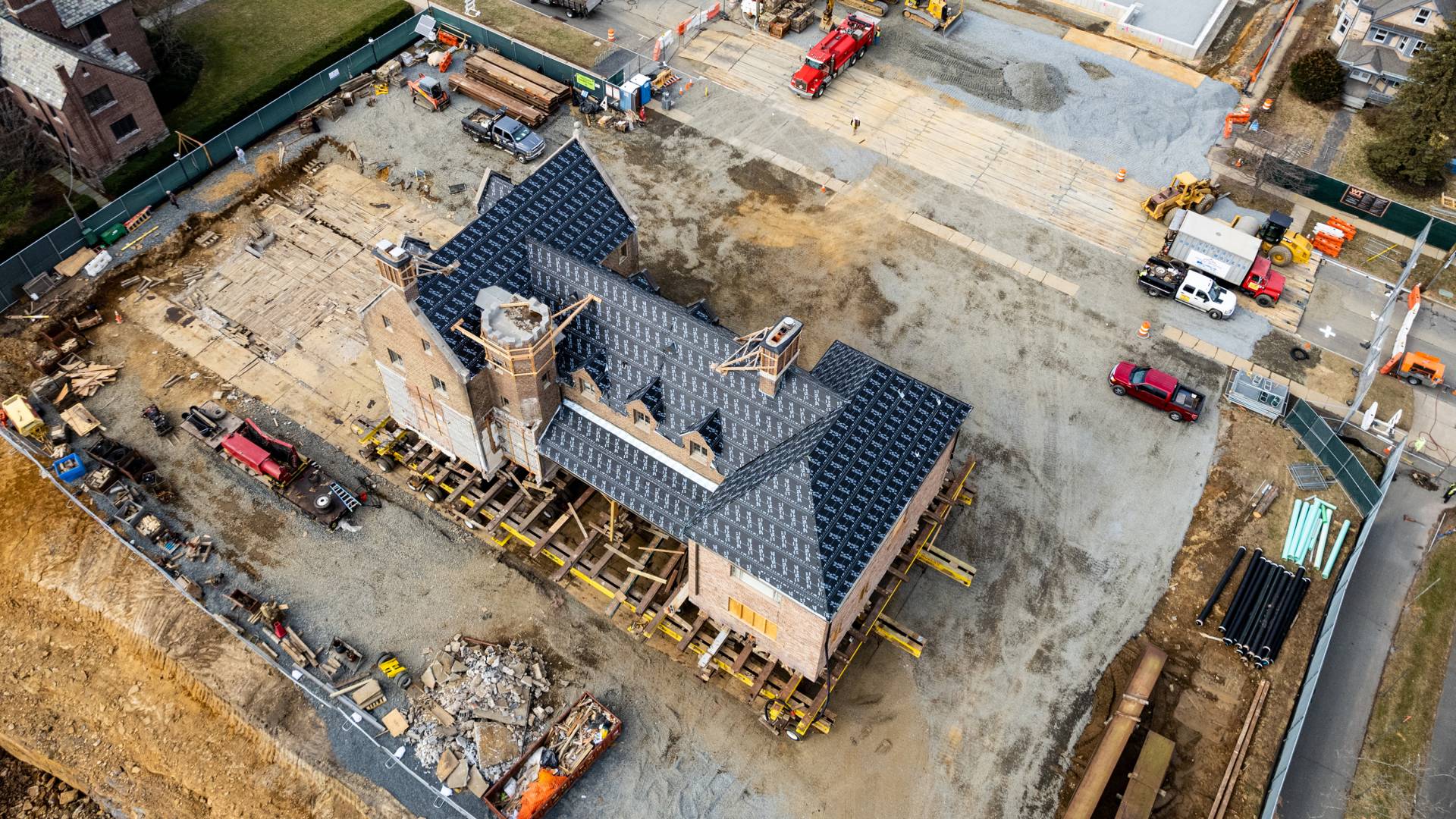The image provides a comprehensive top-down view of a house undergoing remodeling, situated on an empty lot, evidencing its relocation by the visible raised foundation. This foundation elevates the house off the ground, indicating either recent placement or ongoing construction. Surrounding the house is a fenced-off construction site bustling with activity. Numerous vehicles populate the scene, including red pickup trucks, equipment trucks, and what appears to be a bulldozer or forklift in the top right corner. The site is strewn with construction materials: unorganized wood, stacks of lumber, broken bricks, pipes, and metal pieces. The house itself is incomplete, displaying unfinished sides without paint or siding, and a roof bearing black and gray shingles. Adjacent to the house, there are additional scattered materials and another house in the top left corner of the image. The bottom left section of the image shows what looks like a cliff or steep drop-off, adding to the complexity and busyness of the site.